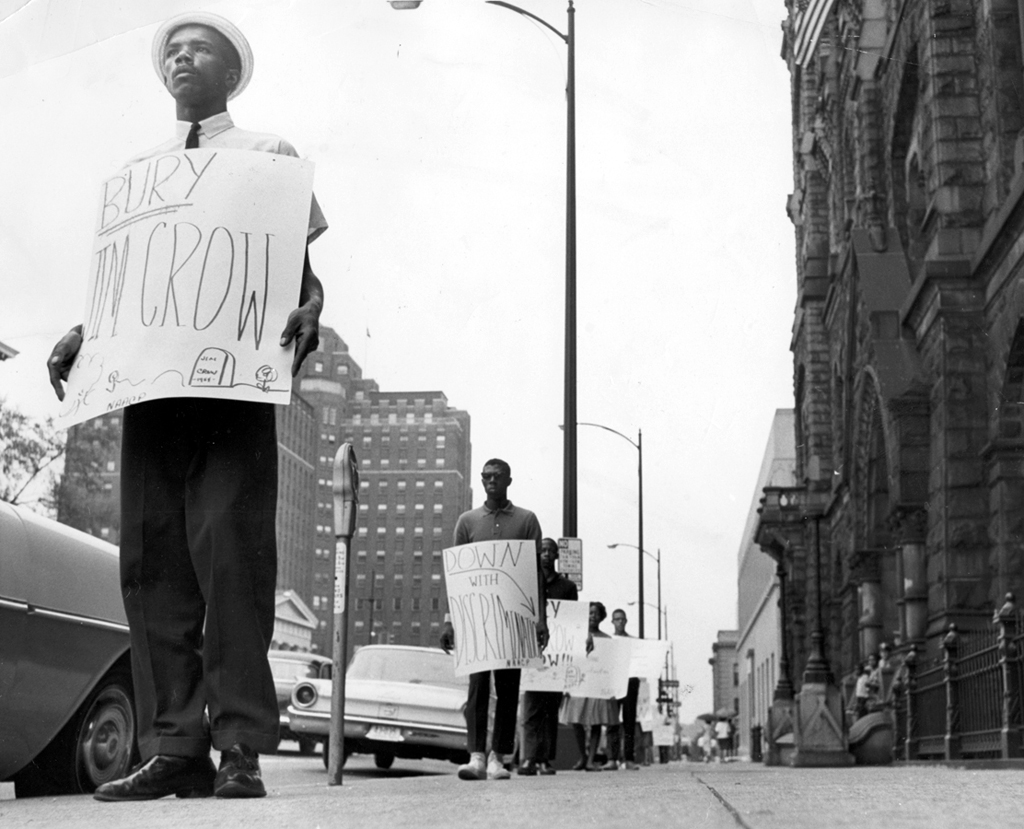In this evocative black-and-white photograph, captured during the 1960s civil rights movement, a group of approximately ten African-American individuals march solemnly down a city sidewalk, each holding handwritten signs that echo their call for justice. The setting is a bustling daytime city street, framed by imposing multistory buildings that hint at office spaces and a gothic-style church, establishing an urban backdrop. 

Prominently, in the top left foreground, stands a black man donning a thin-brimmed hat, a white short-sleeved button-down shirt, a black tie, and dark pants and shoes. He clutches a poignant sign that reads "Bury Jim Crow" accompanied by a sketch of a headstone. Directly behind him, a black man in a gray shirt, dark pants, and light sneakers holds a sign declaring "Down with Discrimination." 

Additional protesters fade into the distance along the sidewalk, their signs partially visible, with one sign showing the letters "Y" and "W." Among them is a black woman in a dress, and more demonstrators whose details blur into the background. Notably, two women, detached from the marching line, walk away holding umbrellas, adding a fleeting normalcy to the tense scene.

Parking meters and vintage cars from the 1950s and 1960s, including a white car and older sedan, line the street. Overhead, a set of streetlights punctuate the gray sky, harmonizing with the vertical lamppost that runs through the center of the square photograph, anchoring the visual narrative of a community united in silent, steadfast protest for civil rights.